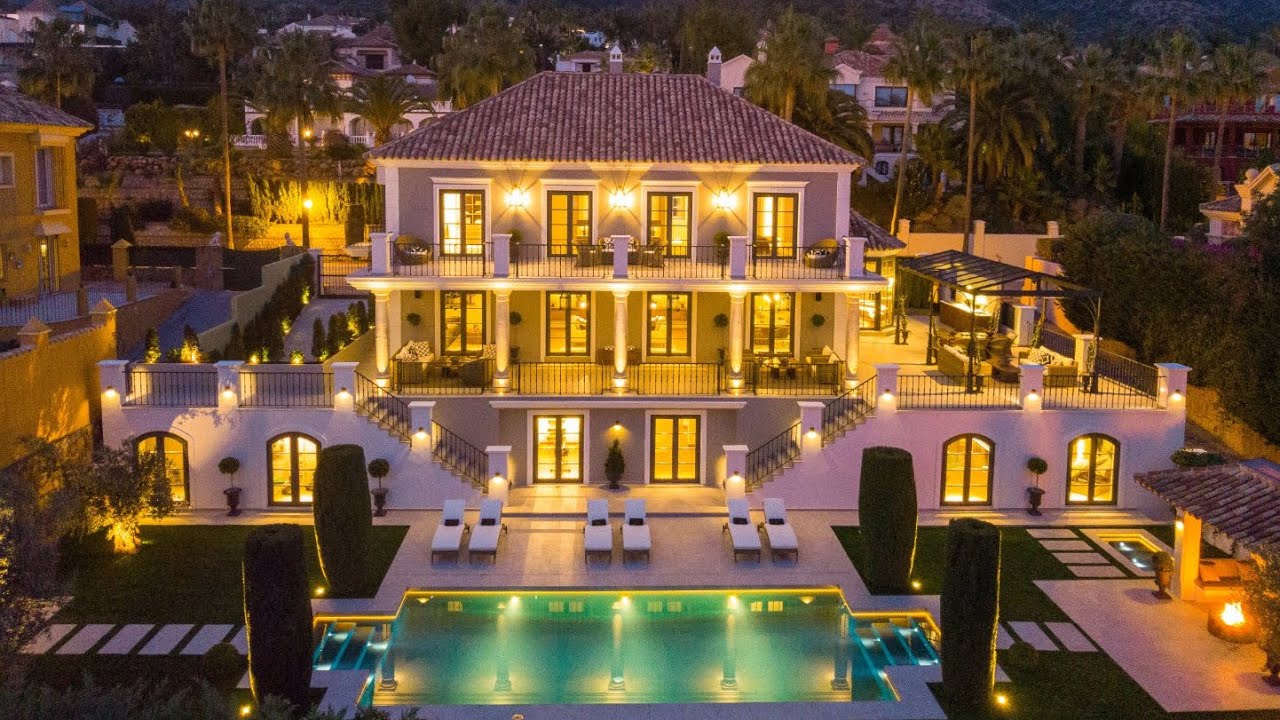This photograph captures a large, three-story mansion bathed in the soft light of dusk. The mansion, predominantly light gray with white accents and a brown, tiled roof reminiscent of clay pottery, is strikingly illuminated by golden glowing lights mounted along its exterior. The lower right corner of the image showcases a lit fire pit beneath an open-sided shelter, adding a cozy ambiance. In front of the mansion lies a centrally located, brightly lit swimming pool, surrounded by six white lawn chairs and flanked by luxuriant greenery and hedges. Two grand staircases lead up to expansive decks on either side of the bottom story, which is broader than the upper ones, creating space for an open rooftop patio on the right side. The background features towering palm trees and other large houses, indicating a sunny, upscale area. The mansion's large windows add to its grandeur, offering a glimpse into what could be an opulent vacation home or an exquisite private residence.